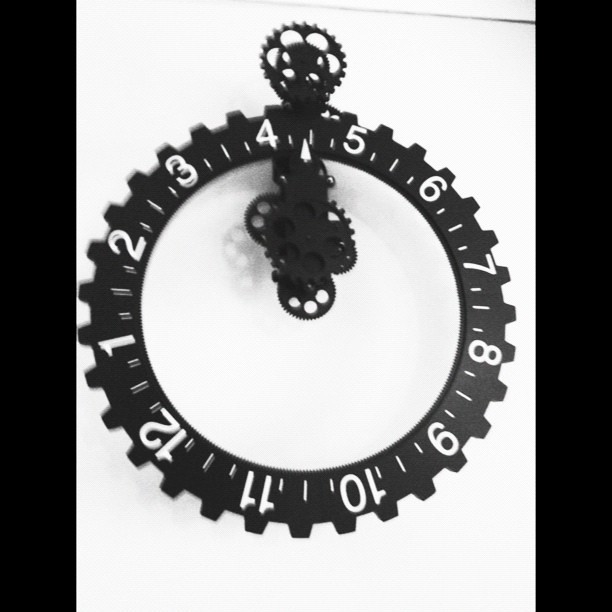This image showcases a distinctive clock face with a mechanical, gear-inspired design. The clock lacks a traditional base, featuring only the face and intricate details. Surrounding the numbers is a circular band giving it a gear-like appearance. Uniquely angled, the clock positions the number 4 at the top, while the number 12 is located at the lower left, indicating a non-standard orientation. The clock hands are designed to resemble gears, with additional gear elements visible above the 4. The center of the clock, from which the hands extend, is a contrasting white, emphasizing the industrial theme of the timepiece.